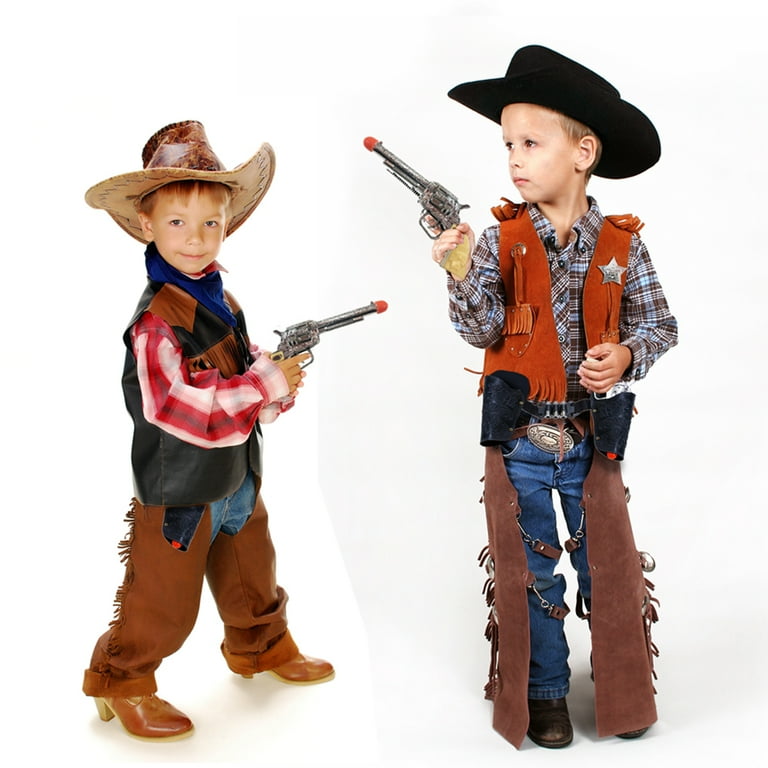In this photograph set against a white background, two young boys are vividly captured in full cowboy attire. The boy on the left, who is shorter, stands facing the camera with his body slightly turned right. He sports a worn brown cowboy hat over light-colored hair, and his dark eyes are fixed on the lens. Dressed in a red and white plaid shirt under a brown and black vest, he also wears oversized brown chaps, which cover his jeans, and reddish-brown boots with yellow heels. In his hand, he holds a silver toy gun pointed towards his taller companion.

The taller boy on the right presents an imposing figure in his black cowboy hat and black boots. His blue and brown plaid shirt complements a brown vest decorated with a prominent sheriff's star. His brown chaps overlay his blue jeans, and he stands confidently with his body facing forward, gazing towards the right, possibly past his younger companion. This boy also holds a pistol, contributing to the sense of readiness for an impending showdown. Both boys, likely around five or six years old, are decked out in what appears to be Western-themed gear, complete with toy Colt Peacemaker guns, making them look adventure-ready cowboys amidst their imaginative play.